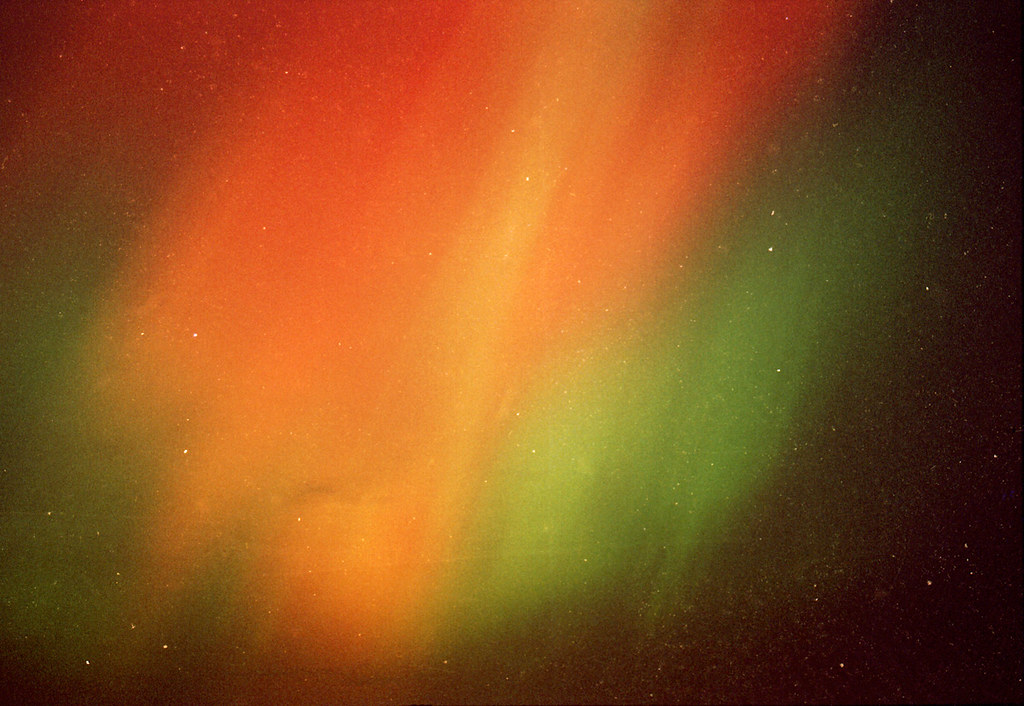The image captures a breathtaking aurora, likely the Aurora Borealis, against a backdrop of a starry night sky. The aurora stretches predominantly across the top left and extends towards the middle right part of the photo, occupying nearly 80% of the image. The colors of the aurora transition smoothly from vibrant red at the top left, blending into shades of orange and yellow in the center, and finally into a deep green moving towards the bottom right. The ethereal nature of the aurora allows stars to be faintly visible through its translucent colors, adding a sense of depth and wonder. The edges of the image, particularly the bottom right, feature a black sky speckled with white stars, enhancing the contrast with the luminous colors of the aurora. The scene is reminiscent of a celestial light show, blending the beauty of natural phenomena with an almost artistic quality.